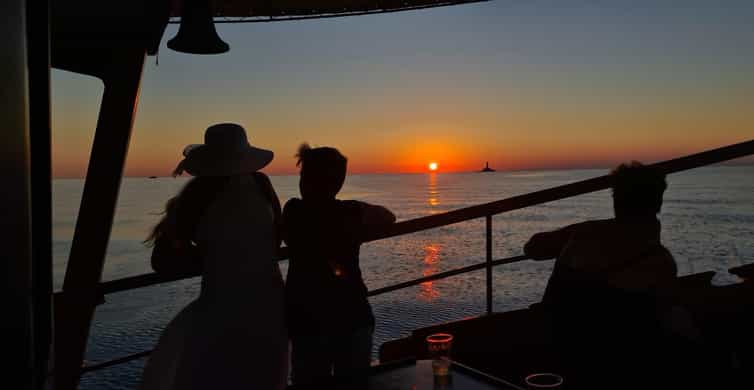The photograph captures a serene sunset scene, moments before the sun dips below the horizon over a large body of water. The upper half of the image showcases a gradient sky, transitioning from a dark blue at the top to a blend of orange and pink near the horizon. The small, glowing orange sun is positioned just above the water's surface, slightly left of center. 

In the foreground, three people are seen from behind as dark silhouettes. They are standing and seated along a diagonal railing that stretches from the bottom left to the center right of the image. The group comprises a woman and a young boy standing with their elbows propped on the railing, and a seated man to the right. They appear to be on a wooden boat dock, identifiable by the wooden structure and railing. To the upper left, a bell hangs, contributing to the maritime setting. 

A table with glasses is partially visible near the observers, suggesting a moment of quiet conviviality as they take in the sunset. Far in the distance, a ship or possibly a lighthouse is silhouetted against the vibrant backdrop, adding depth to the composition. The overall scene is rendered in a clear, colorful realism, capturing the tranquil and contemplative mood of the setting sun.